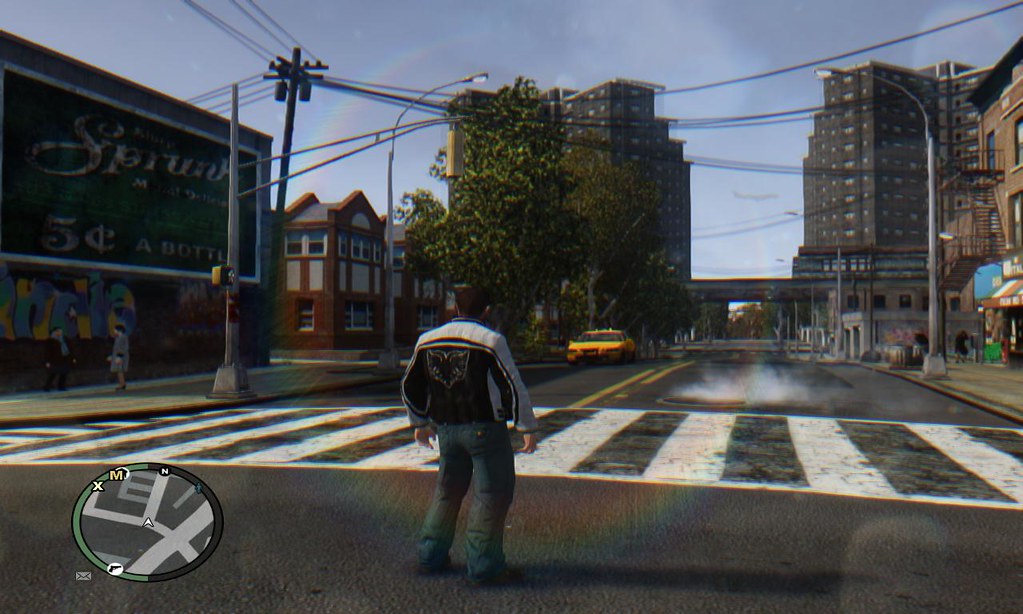In this vivid and detailed image, a person stands at the center of an intersection, reminiscent of a video game setting. Positioned in front of a crosswalk, they are attired in jeans and a distinctive black jacket characterized by gray shoulders and sleeves, adorned with an outlined image of a ram on the back. Their dark hair is visible as they face the viewer amongst the urban scene. Nearby, steam billows from a manhole cover, adding to the atmospheric details. Further down the street, a yellow taxi can be seen approaching, while a building with an advertisement boasting "5 cents a bottle" adds a retro touch to the setting. Sidewalks are dotted with a few pedestrians, and the background reveals a cityscape complete with additional buildings, scattered trees, a bridge or highway, and power lines. In the left corner, within a circular frame, a compass-like or directional indicator provides a further hint at the navigational elements typical of video game interfaces.